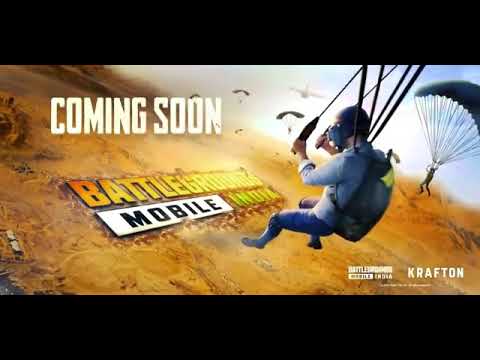This advertisement for the upcoming mobile video game "Battleground Mobile India" is dominated by a CGI animation of several parachutists descending toward a barren, brown landscape with a small patch of blue water in the lower left corner. The most prominent figure in the scene is a man in a light blue button-up shirt, dark blue pants, and boots, with knee pads and a sort of mask over his face. His parachute isn't visible, only his rigging gear, while in the background, you can see five other parachutists with their parachutes fully deployed. The sky is mostly clear with a few clouds, and a distant plane is faintly visible. The text "Coming Soon" is boldly displayed in white at the top left corner, while diagonally across the center, the words "Battleground Mobile India" are embedded into the ground in a combination of white block and yellow letters. The lower right-hand corner features the brand name "Crafton" in small uppercase white font, accompanied by a smaller logo. The advertisement is framed with plain black borders, providing a stark contrast to the vibrant in-game scene.